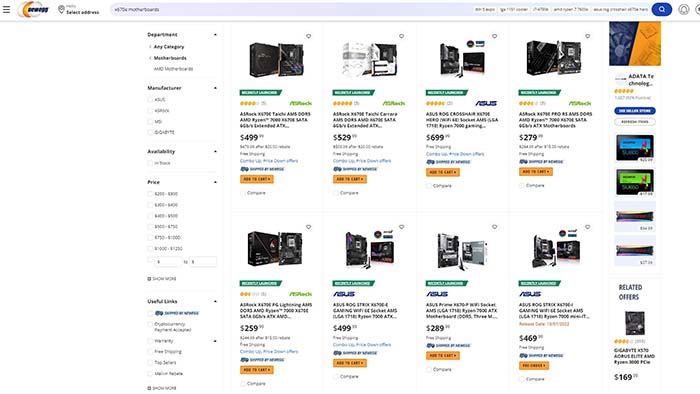The image features a user interface displayed against a white background. At the top of the screen, three black lines are visible, accompanied by a small double circle with gold accents and tiny black print. Adjacent to these elements is a search box with a blue icon containing a magnifying glass. Additionally, various other icons are spread across the top.

On the left side of the image, there are sections detailing product descriptions, departments, availability, and prices, complete with arrows for navigation. The central area showcases eight different product listings, each with a green arrow beneath it. The prices of these products are as follows: $4.99, $5.29, $6.99, and $2.79 on the first four items, and $2.59, $4.99, $2.89, and $4.69 on the next four. All products feature a yellow button beneath their prices.

To the right, there's a dual-colored square, split between blue and yellow, with a blue button and a white button underneath. Below this section, a blue screen and a green screen are displayed side by side. Further down, two light blue boxes appear, followed by a section titled "Related Offers" listing a product priced at $169.99.